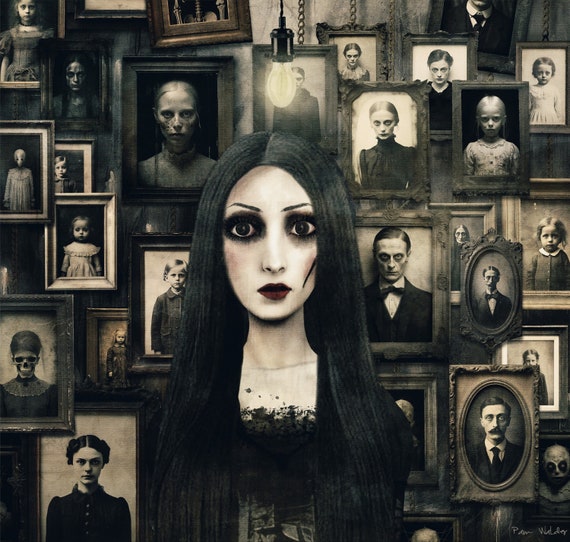The image depicts a stylized, almost photorealistic, yet exaggerated fan art of a gothic woman reminiscent of Wednesday Addams. She stands out with her pale white skin, long straight black hair parted down the middle, and large black eyes heavily lined with dark makeup. Her lips are a striking dark crimson red, and she dons a black dress or blouse adorned with lace. Her face features a distinctive scar or cut on her right cheek, adding to her somber and eerie demeanor. Above her hovers a single bare light bulb, casting an ominous glow over the scene.

Behind her, a wall is adorned with around twenty vintage-looking, black-and-white portraits in various frames. These portraits depict people with haunting, blank eye contact, some with sunken eyes or visible wounds, contributing to the overall spooky, horror movie ambiance. One particularly macabre portrait even shows a person with an exposed skull for a face, while others resemble typical Victorian era photographs of individuals and children. The entire composition, with its collage-like arrangement of framed images and the woman's gothic appearance, exudes a creepy, Halloween-like atmosphere.